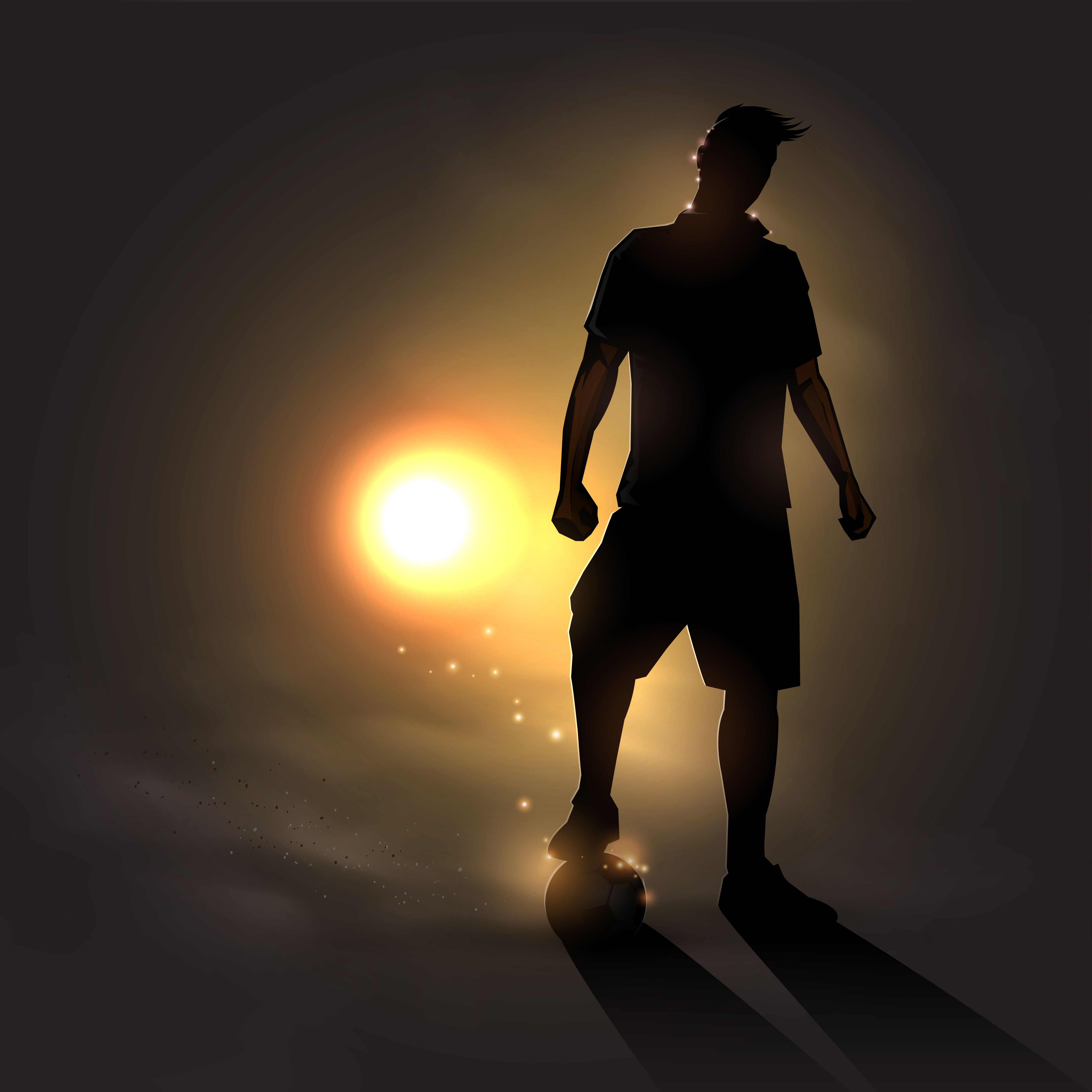In the digital artwork, a shadowy figure of a man is positioned with one foot resting on a round ball. The background of the image is predominantly black, giving a dramatic contrast to the central bright circle that appears like a glowing sun. This sun-like circle is outlined in orange and radiates white, sparkling lights from its bottom, which seem to flow toward the ball under the man's foot. The man’s form is a featureless silhouette, casting a shadow due to the bright light behind him. His short hair is distinguishable, and he is dressed in a collared, short-sleeved shirt with shorts that reach his knees. His arms are extended downward with clenched fists at his sides. The overall effect of the image creates a powerful, almost celestial atmosphere, emphasizing the glowing sun-like orb and the surrounding sparkles.